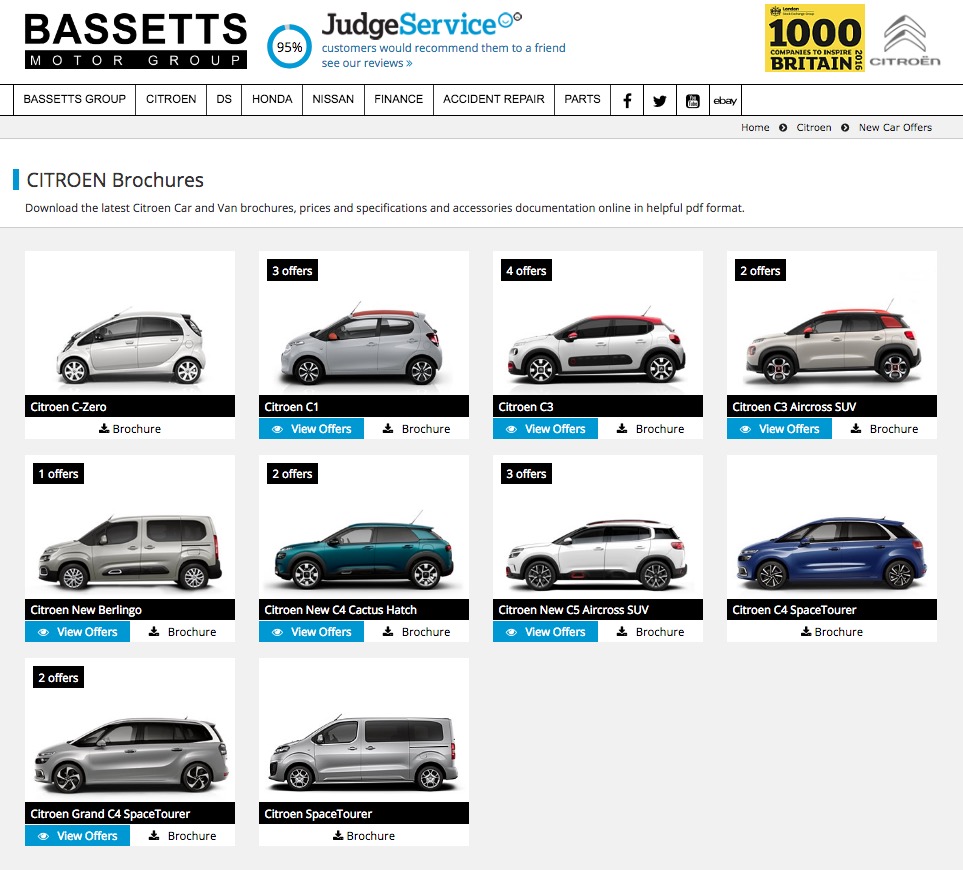This vertical image captures a detailed view of a webpage, likely optimized for display on various devices including desktops, laptops, and smartphones. The background seamlessly blends with the white of the computer screen in certain areas. Dominating the header on the left is the text "BASSETS" in bold uppercase black font, underlined by a black rectangular box with "Motor Group" inscribed in white within it. Adjacent to this, a blue circle prominently displays "95%" indicating a high customer recommendation rate by Judge Service, suggesting that those customers would recommend the company to their friends. A clickable link invites viewers to see further reviews.

On the upper right, there's a bright yellow section that reads "1000 Companies to Inspire Britain" in black text, accompanied by a Cintron icon. Moving back to the left, a series of clickable tabs are present, including options like Basset Group, Cintron, DS, Honda, Nissan, Finance, Accent Repair Parts, alongside various social media icons.

Beneath this, on the upper right, you'll find the Home button, Cintron, and New Car Offers. On the left again, a small vertical blue rectangle is marked beside the text "Cintron Brochures" in black. Below these items, the webpage features images of vehicles, detailing their names, the number of offers available for each, and clicking options for more information.